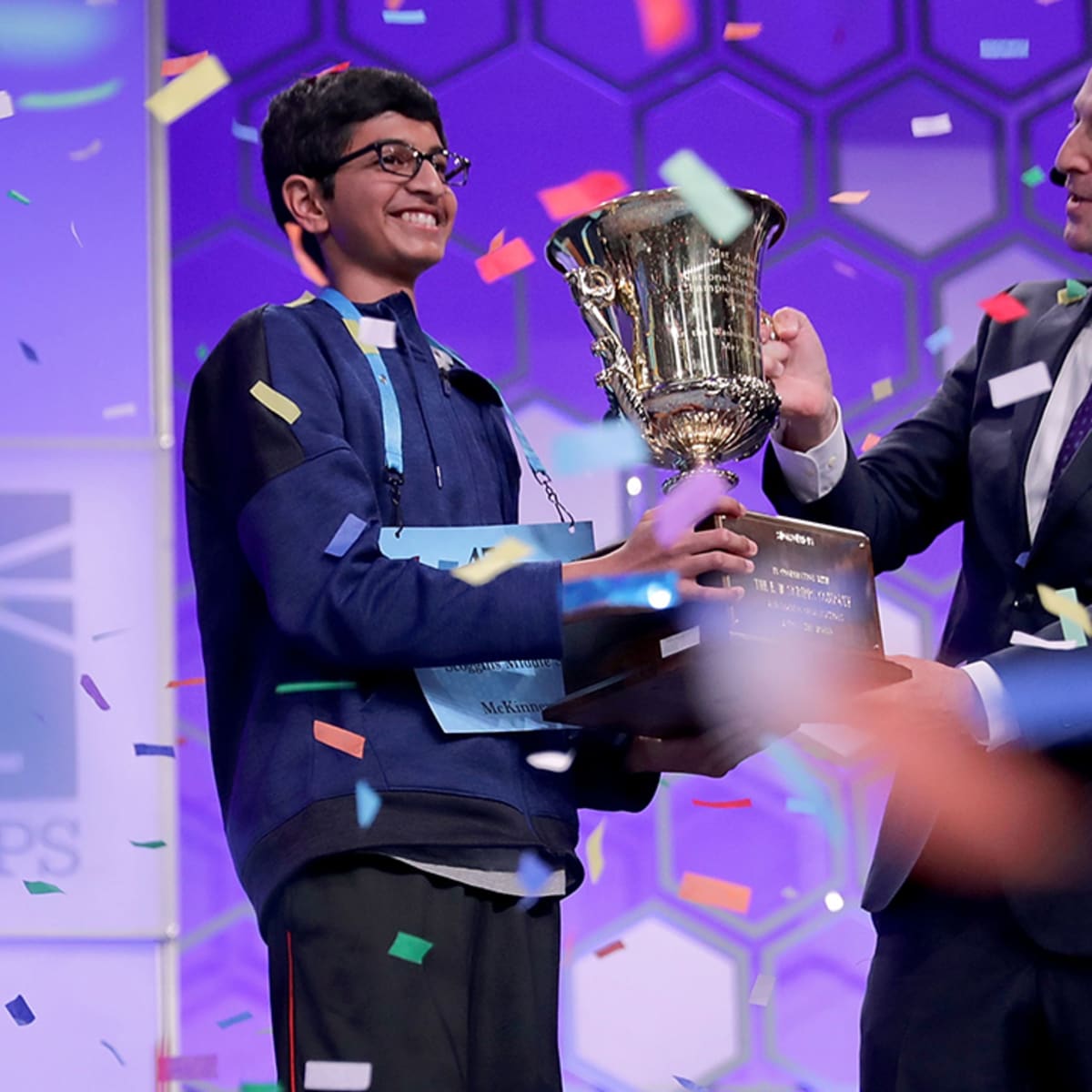In this vibrant and celebratory rectangular color photograph, we see a young boy of Asian descent, likely from India, joyfully receiving a large trophy from an older gentleman whose arms and hands are visible off to the side. Grinning broadly, the boy's eyes shine behind his black-rimmed glasses, and his black hair is neatly styled. He is smartly dressed in a blue jacket with black accents, paired with black pants. The scene is bursting with energy as red, yellow, green, blue, and white confetti rains down, encapsulating the moment of victory and excitement. The child stands to the left, with the man helping to hold the trophy to the right. Although the text on the trophy is unreadable, the trophy has a prominent square base and is clearly significant. Set against a dark blue background, this image captures the essence of a triumphant and joyful event, frozen in time with high-quality clarity.